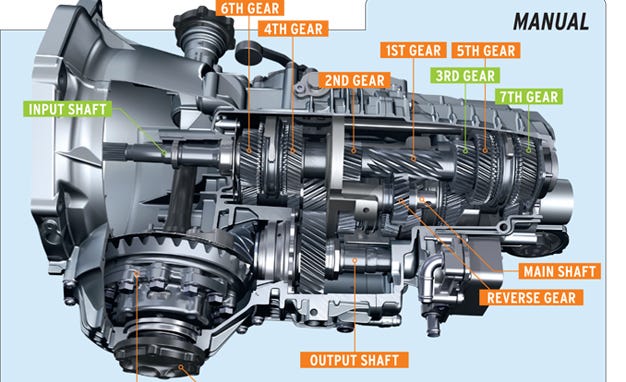This is an illustrated page from a manual for a mechanical system, likely an engine or transmission. The top-right corner of the page prominently features the word "manual." The diagram on the left side of the page depicts a detailed internal view of the system, resembling the inner workings of a manual pencil sharpener. The item is primarily gray, set against a light blue background, with labels highlighted in either orange or green rectangles with white text. The green labels denote the input shaft, third gear, and seventh gear, while the orange labels indicate the sixth gear, fourth gear, second gear, first gear, fifth gear, main shaft, and reverse gear. The layout of the diagram shows a tapering shape from left to right, with a series of gears and mechanical components such as screws and grinding wheels. The illustration provides a comprehensive view of the arrangement of different gears and shafts within the system, giving insight into the intricate mechanical details that would typically be hidden within an assembled unit.